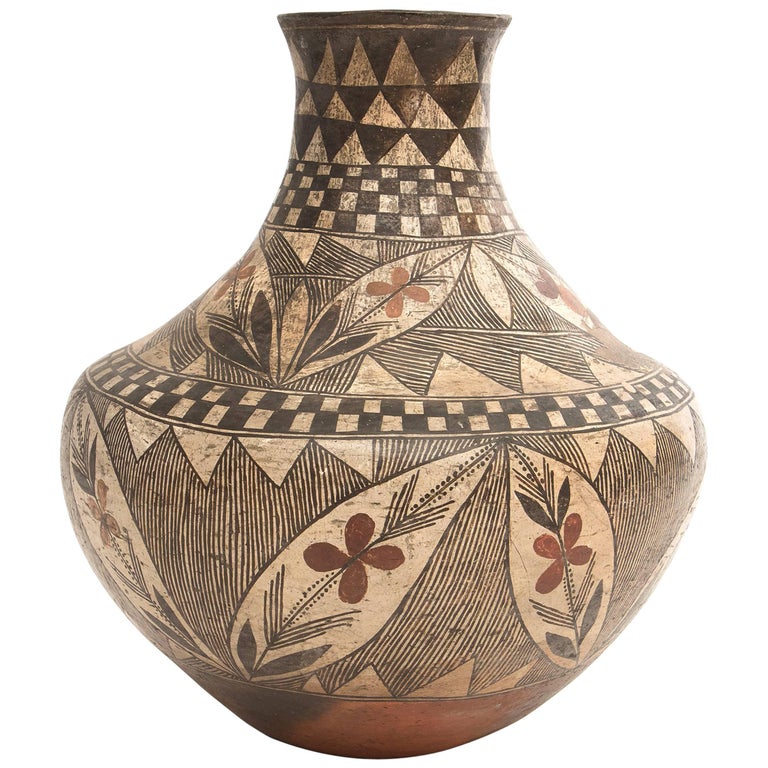This is a photograph of an antique terracotta vase prominently displayed against a white or transparent background, likely intended for commercial purposes. The vase features a distinctive shape, widening around its midpoint before tapering dramatically towards its neck. The lower section of the vase is plain brown terracotta without any design. Above this, the vase showcases intricate designs: starting with a black and white triangular pattern near the top, followed by a checkerboard motif. Moving further down, you see artistic depictions of leaves adorned with small dark brown flowers, arranged in a pattern reminiscent of arrows pointing upwards. These elements reappear just below the midpoint, followed by another band of the checkerboard pattern. The vase demonstrates a traditional, possibly handcrafted aesthetic, characterized by its detailed and repetitive geometric and natural motifs.